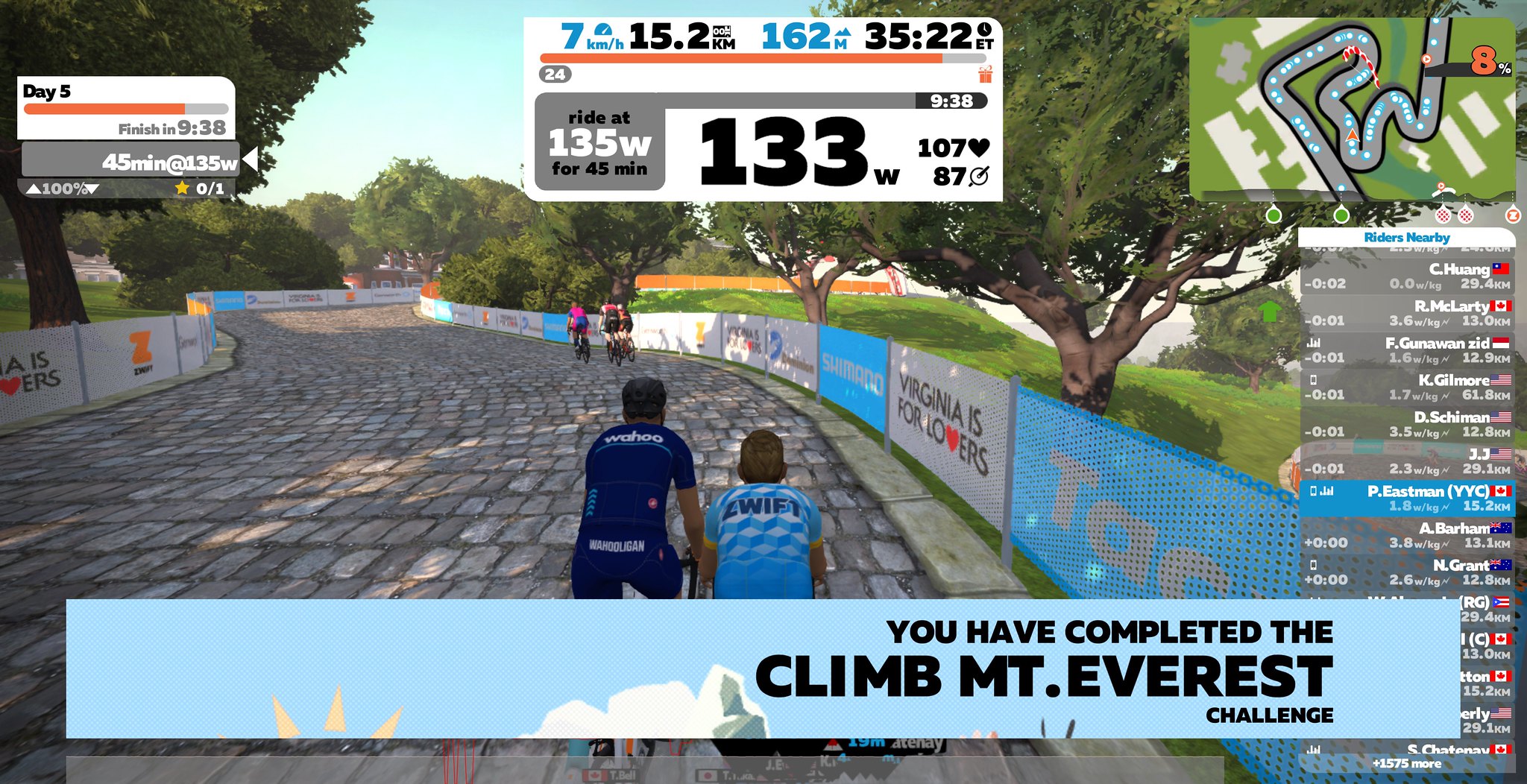In this highly detailed and photorealistic or possibly computer-generated image, the focus is on a racing scene from a video game set on a winding flagstone pathway, flanked by walls. Central to the image are five cyclists: two in the foreground wearing black and light blue jerseys emblazoned with "Ever Who" and "ZWIF," and three in the background dressed in red and black. They appear to be part of a mid-race scenario under a clear, daylight sky.

At the bottom of the image, a banner proclaims, "You have completed the Climb Mount Everest Challenge," while various informational graphics populate the screen. The top left corner displays a status readout: "Day 5, finish in 9:38:45 minutes at 135W, 100%, 0/1." Another prominent graphic provides in-depth race details: "7 kilometers per hour, 15.2 kilometers, 162 meters, 35:22 ET, 24 riders at 135W for 45 minutes, 133, 9:38, 107, hot, W87."

On the right side, a radar icon and track information offer additional context on race positioning. Notable signs along the pathway include "Virginia is for lovers" and a partially obscured sign featuring a "Z." The bottom banner details nearby riders’ metrics, displaying various names, national flags, power-to-weight ratios (W/KG), and distances covered, such as "Rick McCloudy," "K Gilmore," and "Pete Eastman."

The vibrant scene is a symphony of light blue, yellow, white, gray, green, orange, red, and black, capturing the excitement and intensity of a cycling race in a simulated outdoor setting.